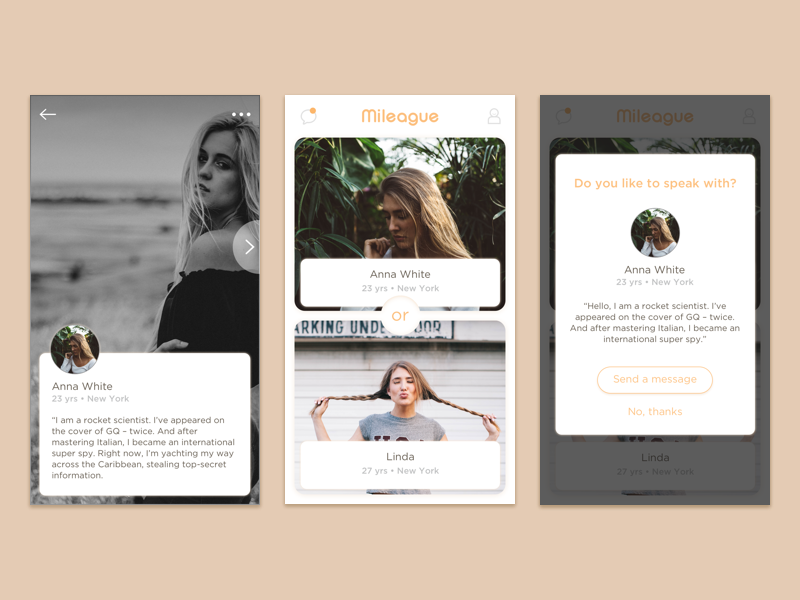The image is a compilation of three screenshots from a dating site, displayed side-by-side. 

The first screenshot predominantly features a black and white photo of a woman with long hair, glancing over her shoulder. Beneath this image is her profile heading, which reads "Anna White, 23 years, New York." Her whimsical and adventurous profile description states: "I'm a rocket scientist. I've appeared on the cover of GQ twice. After mastering Italian, I became an international super spy. Right now, I'm yawning my way across the Caribbean, stealing top-secret information."

The second screenshot, titled "Mileage," includes two distinct photos. The first is another picture of Anna White, this time standing in a grassy area surrounded by high green bushes. Next to her, there's an image labeled "Linda, 27 years, New York," depicting a woman making duck lips and holding out her braids.

The final screenshot to the right contains a pop-up box asking, "Do you like to speak with?" under which Anna White's profile picture is displayed again. Her descriptive words are repeated underneath with options to either send her a message or select "No, thanks."